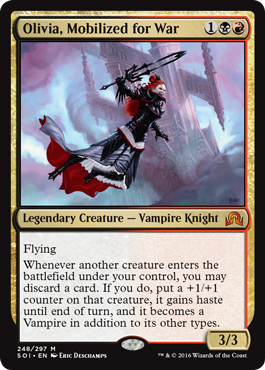This image depicts a trading card with intricate and detailed artwork. Encased in a complete black border, the card features an elegant gold border wrapping around its upper section—the left, right, and top sides—encircled in black. At the top of the card, within the gold bordered area, the name "Olivia, Mobilized for War" is clearly printed, alongside a symbol denoting the number one, a skull icon, and a gold icon.

The central visual of the card presents a striking character set against a stormy blue background, implying tumultuous weather. The character is a soldier with vivid red hair, dressed in a black coat which transitions into a white section at its base. She is adorned in a black and white dress, complemented by black boots, and a striking red and black cape that billows behind her. She wields a formidable black sword, emphasizing her readiness for battle.

Beneath the artwork, in gold text, the card identifies the character as a "Legendary Creature – Vampire Knight." Below this title is a white box containing crucial gameplay mechanics detailed in black writing: "Flying. Whenever another creature enters the battlefield under your control, you may discard a card. If you do, put a +1/+1 counter on that creature. It gains haste until end of turn and becomes a Vampire in addition to its other types."

At the bottom of the card, also in gold text, are the stats "3/3," denoting the creature's power and toughness. There is additional white text in a black box at the very bottom of the card, though this text is unreadable in the provided image.